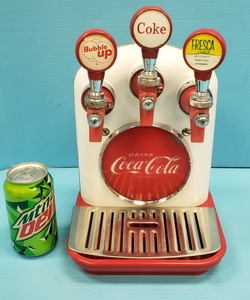The image depicts a vintage-style soda dispenser, reminiscent of the 1950s or 1960s. The dispenser is predominantly white with rounded edges, featuring a central circular logo bearing the iconic Coca-Cola emblem. At the top of this nostalgic machine, there are three lever-like handles used for dispensing drinks, each adorned with different brand logos: Bubble Up on the left handle, Coca-Cola in the center, and Fresca on the right. Below these handles, there is a grated drink catcher, similar to those seen in fast food restaurants. Adjacent to the dispenser is a modern-day can of Mountain Dew, offering a size comparison, revealing that the dispenser is about twice the height of the can. Both items are set against a light blue backdrop, with the surface beneath the dispenser being an even lighter shade of blue. The scene suggests a product showcasing, possibly for sale, highlighting both the vintage aesthetic and the compact size of the soda dispenser.